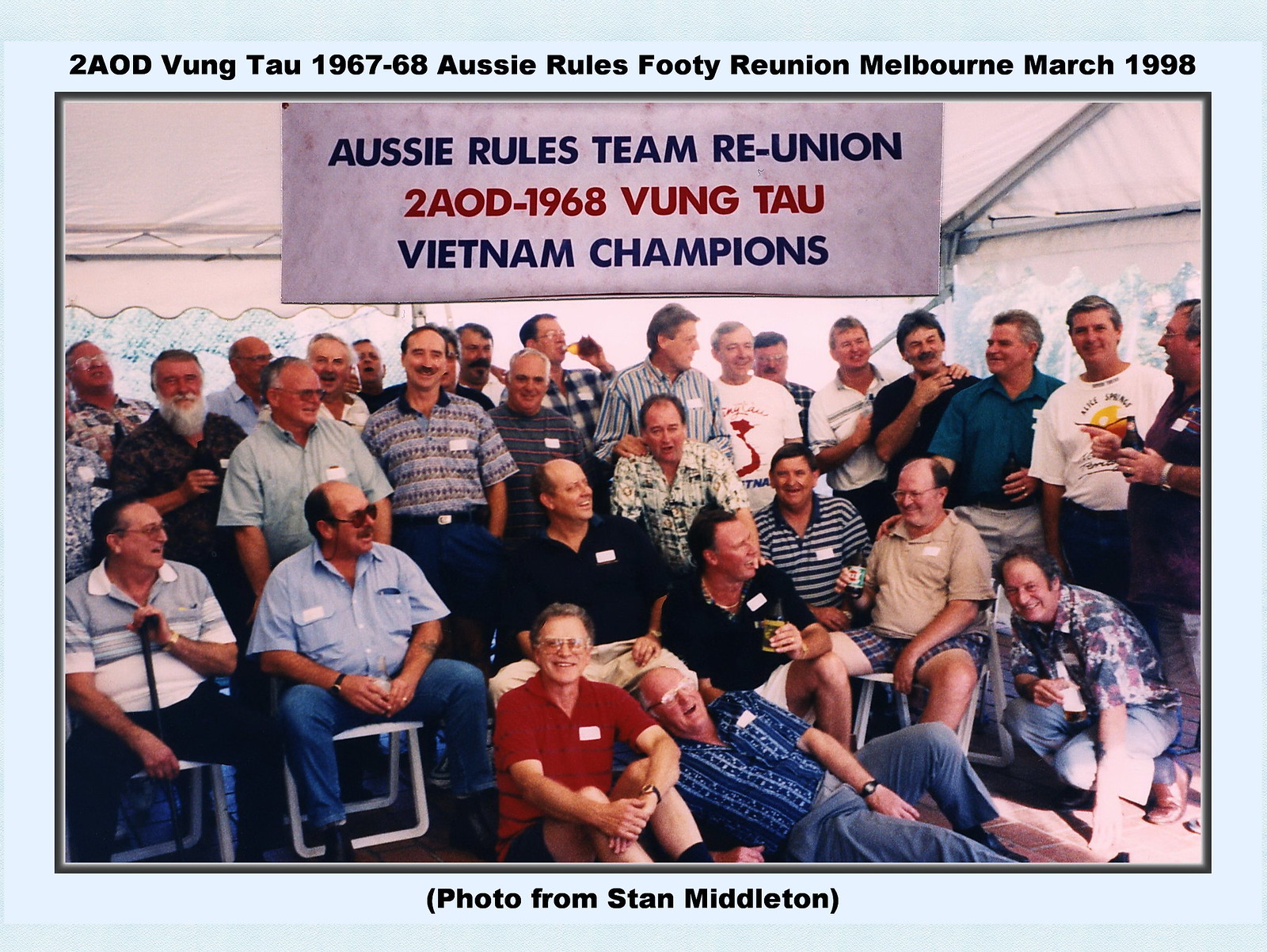A photograph captures a large group of men at a reunion, and is set against a light blue background with a white tent overhead. The event is titled "Aussie Rules Team Reunion 2 AOD 1968 Vung Tau Vietnam Champions," as displayed on a red and blue banner hanging prominently above the group. Additional text at the top of the page reads, "AOD Vung Tau 1967-1968, Aussie Rules Footy Reunion, Melbourne, March 1998." The men, numbering between 20 to 25, display a wide age range from middle-aged to older adults. They are arranged in several rows with a few crouched on the floor, some standing, and others seated, all smiling and engaging warmly with one another. Some of them hold beers and wear name tags on their chests. This joyful gathering is further identified by a note beneath the image, stating "(photo from Stan Middleton)." One notable detail in the front row is a man in red directly looking at the camera, while others appear to be conversing and laughing with each other.